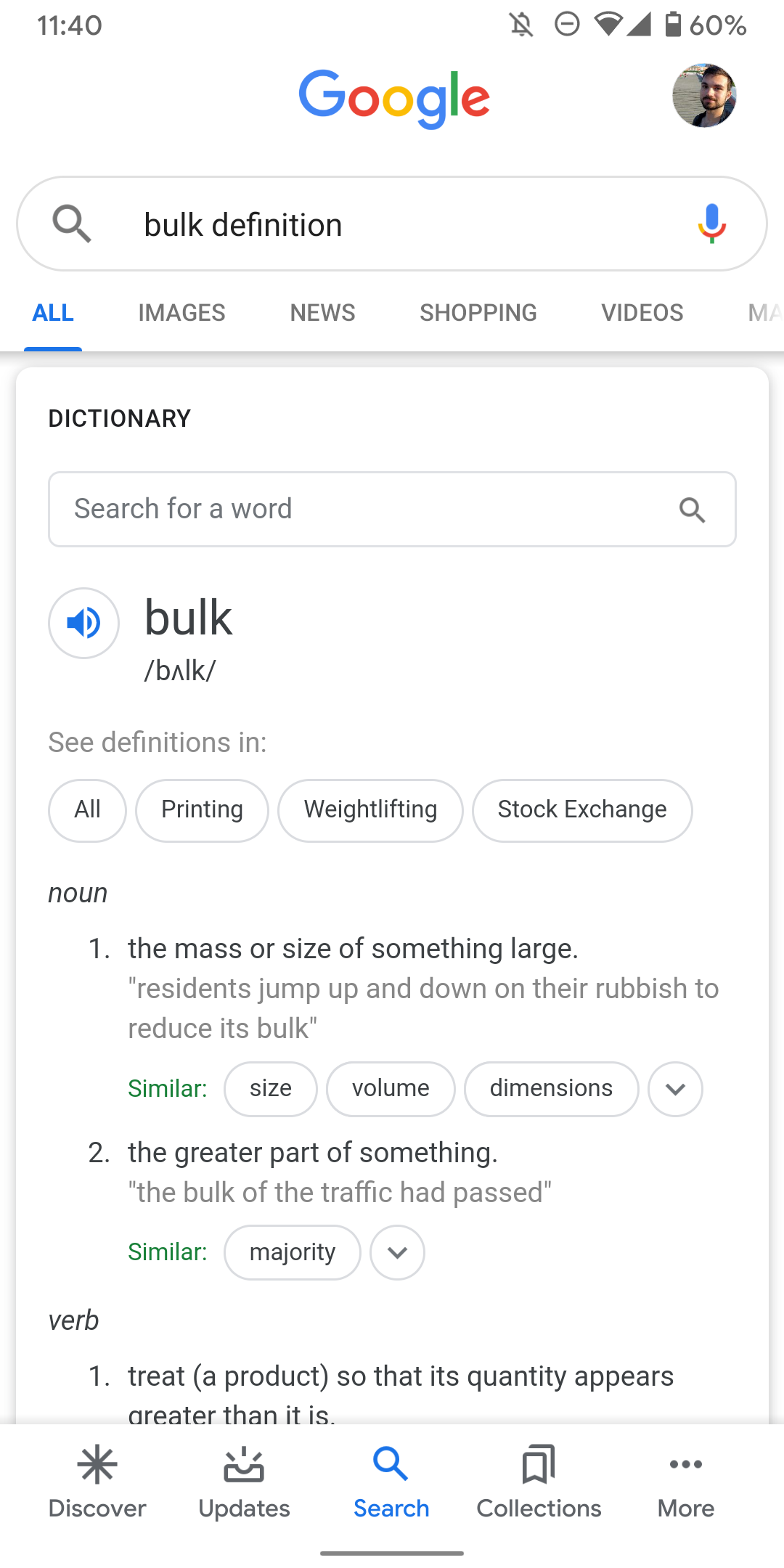This image appears to be a screenshot of a Google search made on a mobile device at 11:40 AM, indicated by a gray timestamp at the top. The notification status shows that notifications are silent, represented by a bell icon with a line through it. Adjacent to the bell icon, there is a circle outlined in gray with a dash in the middle, followed by a WiFi symbol, then a data signal strength indicator, and a battery icon showing 60% charge. Below the battery icon is a circular icon featuring an image of a male.

On the left side at the top, the Google logo is displayed in its traditional colors: the first "G" in blue, the first "O" in red, the second "O" in yellow, the "G" in blue, the "L" in green, and the "E" in red. Below the logo is an elongated search bar where the user has typed "bulk definition," shown in a black font. To the right of the search bar, there is a microphone icon, and to the left, a magnifying glass icon.

Beneath the search bar is a navigational menu with several options. The "All" option is selected, indicated by bold blue text and a blue underline. The other menu options—Images, News, Shopping, and Videos—are shown in gray text.

In the search results area, "DICTIONARY" is displayed in bold black capital letters, indicating the type of content. There is another search query field with a magnifying glass icon on the right for searching a word. Next to this is a gray circle with a white background containing a blue speaker icon, which, when clicked, enables Google to pronounce the word. The word "bulk" is written next to it in bold black lettering.